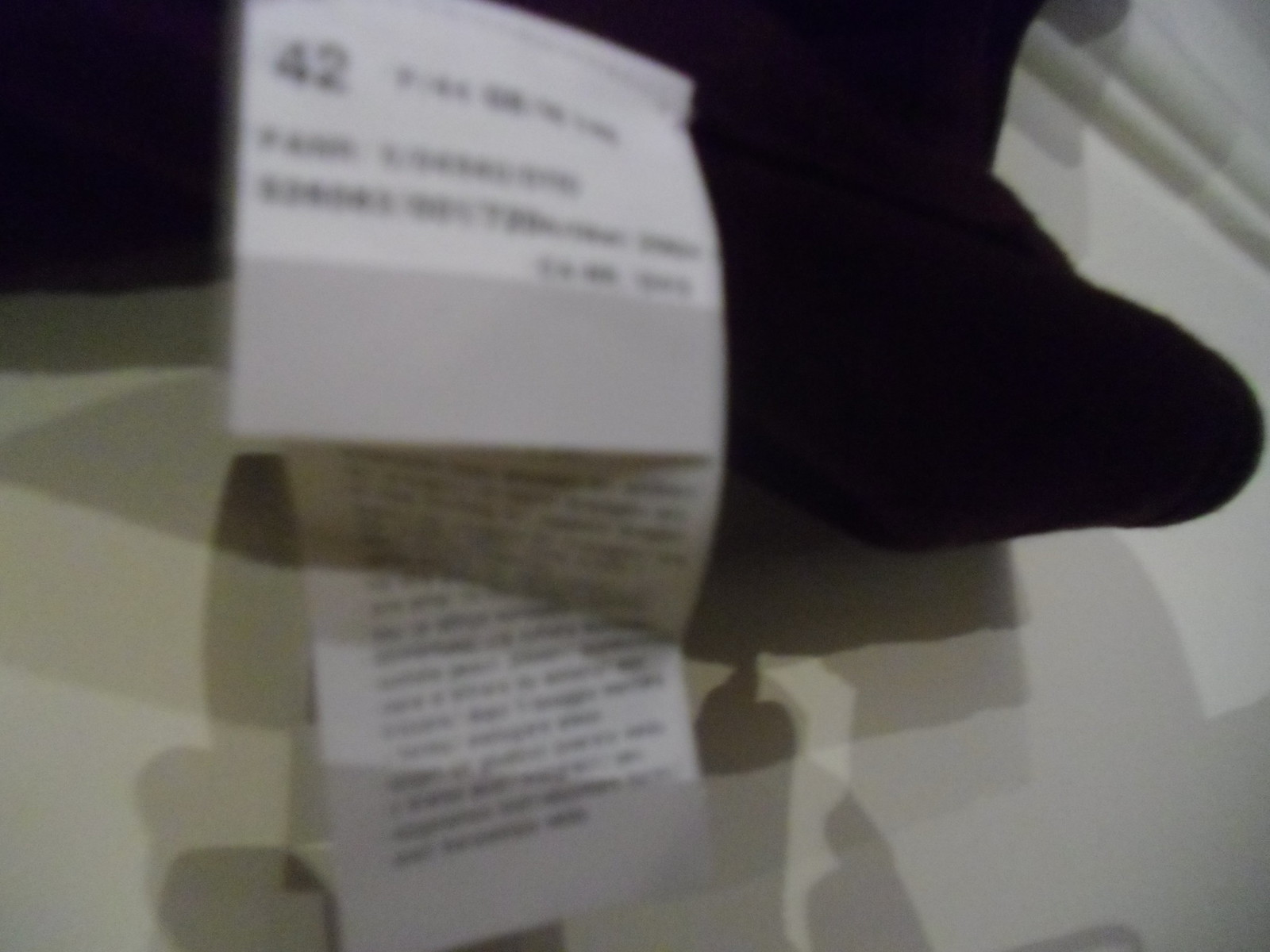This is a blurry photograph taken in low-light conditions, featuring a white label sewn onto a black piece of clothing. The image prominently shows the number 42 in black on the top left corner of this white label. Behind this label, there is a longer white tag with a significant amount of smaller black text, though the exact details are unreadable due to the blurriness. The black clothing curves slightly to the right. The background consists of a beige and gray surface, likely a table, with shadows of the person taking the photograph visible at the bottom.